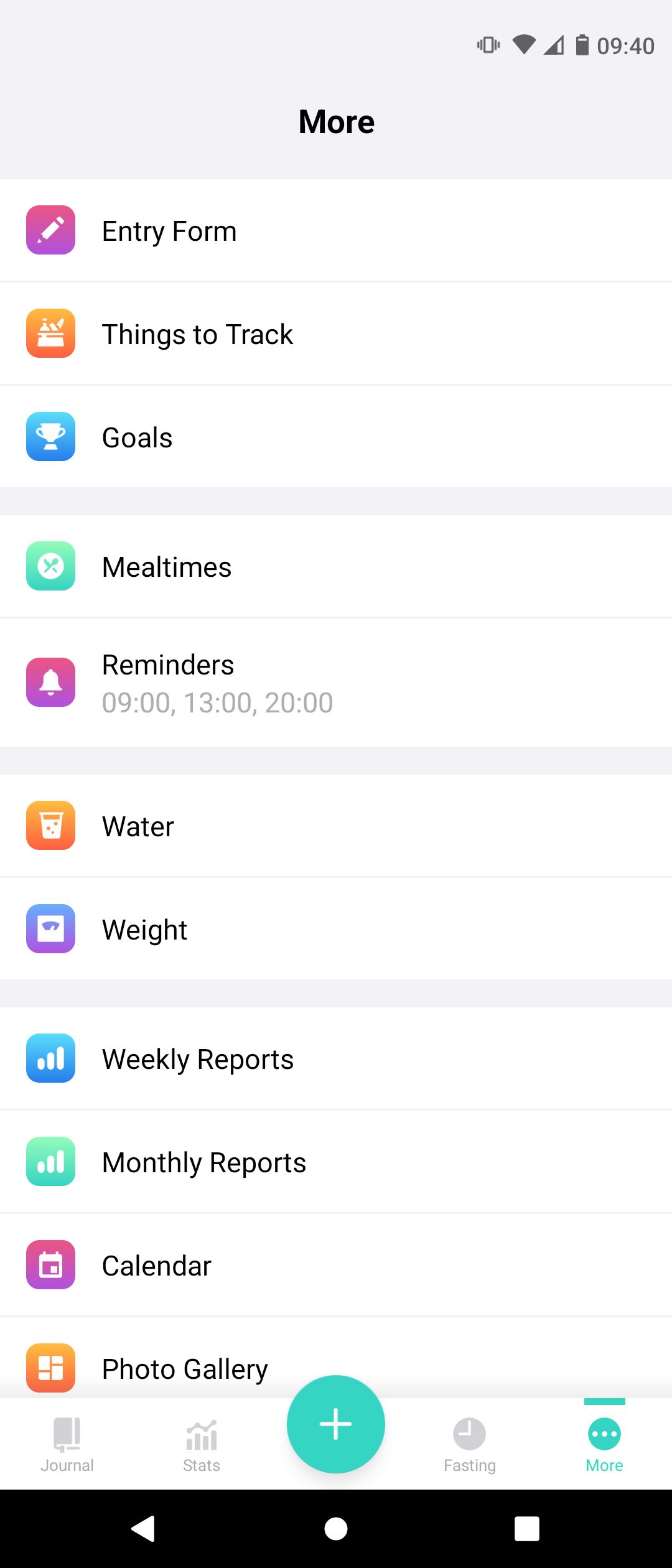This image showcases the user interface of a mobile application on a smartphone. At the top of the screen, the status bar is visible, displaying essential indicators such as Wi-Fi signal strength, network strength, battery level, and the current time. Just below the status bar, there is a "More" option, possibly indicating additional features or settings.

The primary part of the screen is dedicated to various interactive icons and buttons, each designed to serve a specific function within the app. The interface begins with an "Entry Form" button at the top, followed by a "Things to Track" button. Continuing downwards, there is a "Goals" button, each accompanied by distinctive icons for easy identification.

Further down, several more buttons are presented:
- A green button labeled "Meal Times"
- A purple icon for "Reminders"
- An orange icon featuring a water glass for tracking "Water" intake
- An icon resembling a scale for monitoring "Weight"
- Buttons for generating "Weekly Reports" and "Monthly Reports"
- A "Calendar" button
- A "Photo Gallery" button

These features suggest the app is likely intended for personal management, health, or fitness tracking, providing users with a comprehensive suite of tools to monitor various aspects of their daily routine.